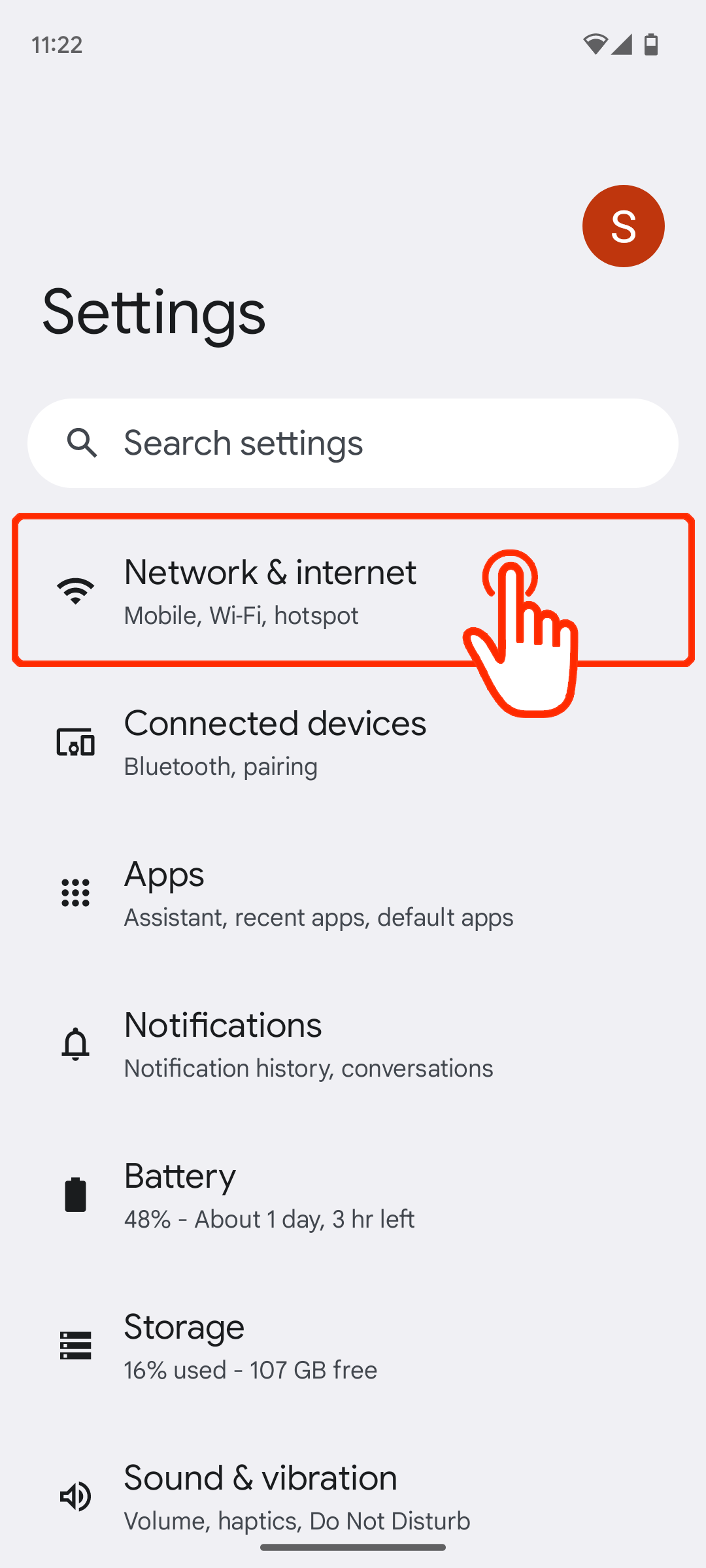This screenshot captures a detailed view of a phone's settings tab on a light gray background. In the upper left-hand corner, there's a timestamp displayed in dark gray text, reading "11:22." The upper right-hand corner features essential status icons, including the battery percentage, cell phone signal strength, and Wi-Fi signal strength. Adjacent to these icons is a white letter "S" enclosed within a red circle.

Beneath the timestamp on the left, the word "Settings" is prominently displayed in bold black text. Directly below this is a search bar designed for navigating the settings. The main section of the screen lists various settings options: "Network & Internet," "Connected Devices," "Apps," "Notifications," "Battery," "Storage," and "Sound & Vibration." 

The "Network & Internet" option is specifically highlighted by a red box drawn around it. An annotation below it reads "mobile Wi-Fi hotspot," accompanied by a hand icon indicating the selection action.

This meticulous layout clearly guides the user toward accessing mobile hotspot settings within their device.